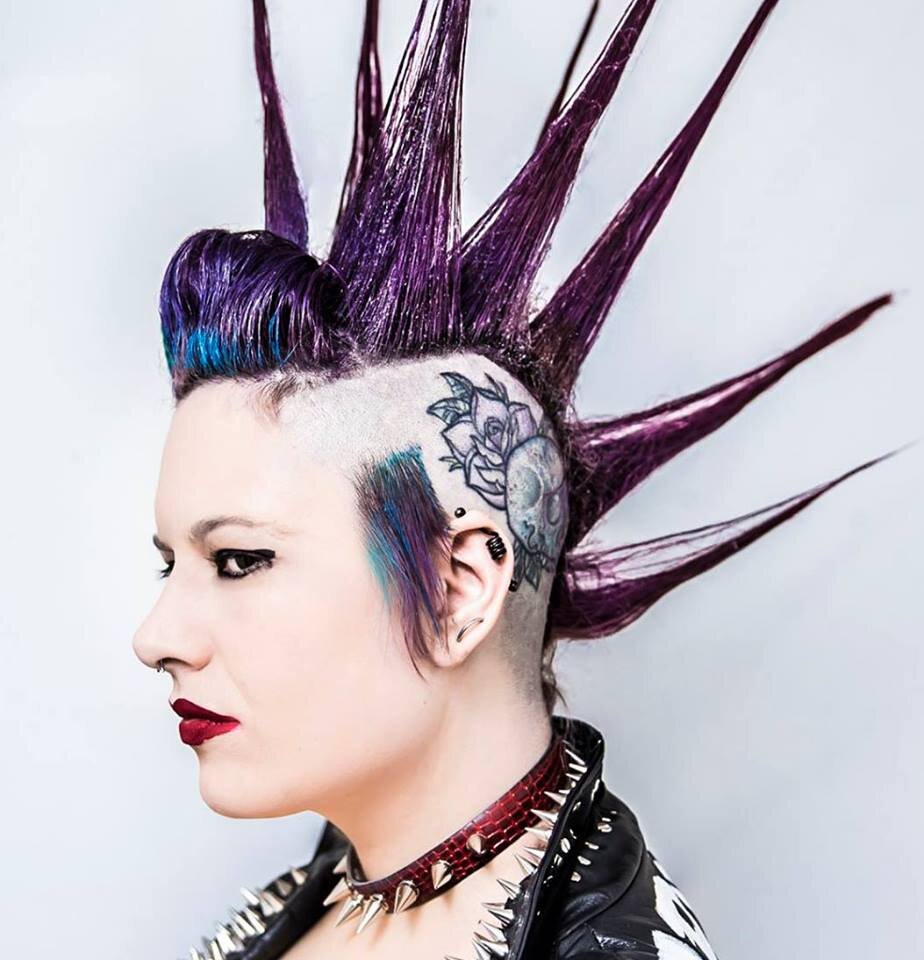The photograph captures a female punk rocker in a side profile view, facing left. Her striking hairstyle features a purple spiked mohawk with up to eight tall, sharp spikes sculpted with wax, extending from the front of her head to the nape of her neck. The sides of her head are shaved, revealing a colorful tattoo of a skull with flowers in hues of blue, yellow, and purple. A small tuft of sideburn hair remains in front of her ear. Her punk aesthetic is further emphasized by her bold makeup, including heavy black eyeliner and bright red lipstick, which gives her a somewhat fierce expression. She wears a red spiked choker around her neck and a black leather jacket adorned with spikes all over the collar, as well as some white lettering on the back, enhancing her rebellious look. The photograph highlights her numerous piercings and the detailed elements of her punk style, making her a compelling and memorable subject.